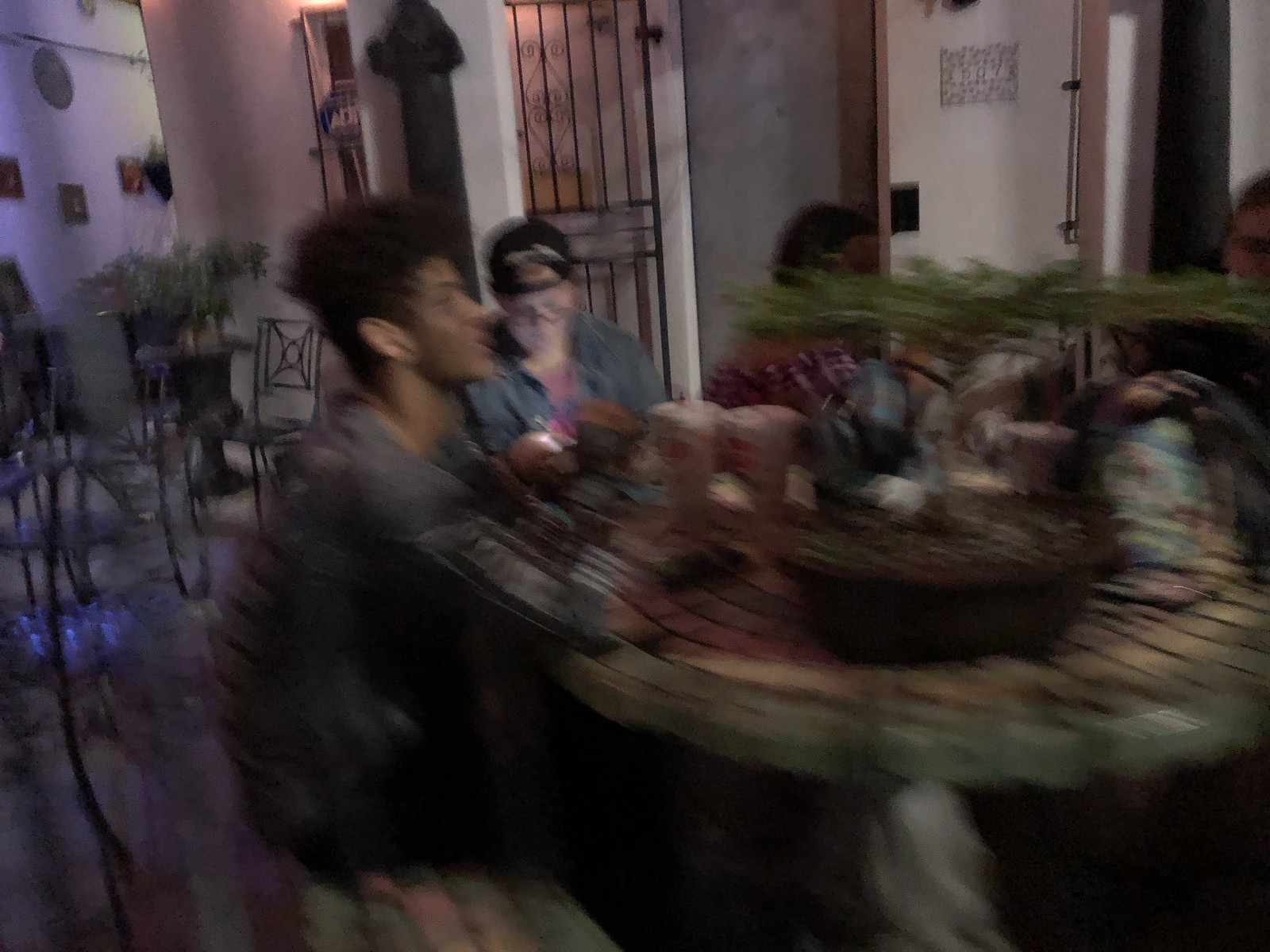A slightly blurry photograph captures a group of people sitting around a round table, constructed from stone-like tiles that match the material of the surrounding benches. The focal point of the image is a person on the left side of the table, facing towards the right, wearing a long-sleeved black shirt with the sleeves somewhat rolled up. Behind the table, three other individuals are also seated, though their features are less distinct due to the blurriness. Notably, one of the people in the background is dressed in a jean jacket. The scene suggests a casual, outdoor social gathering.